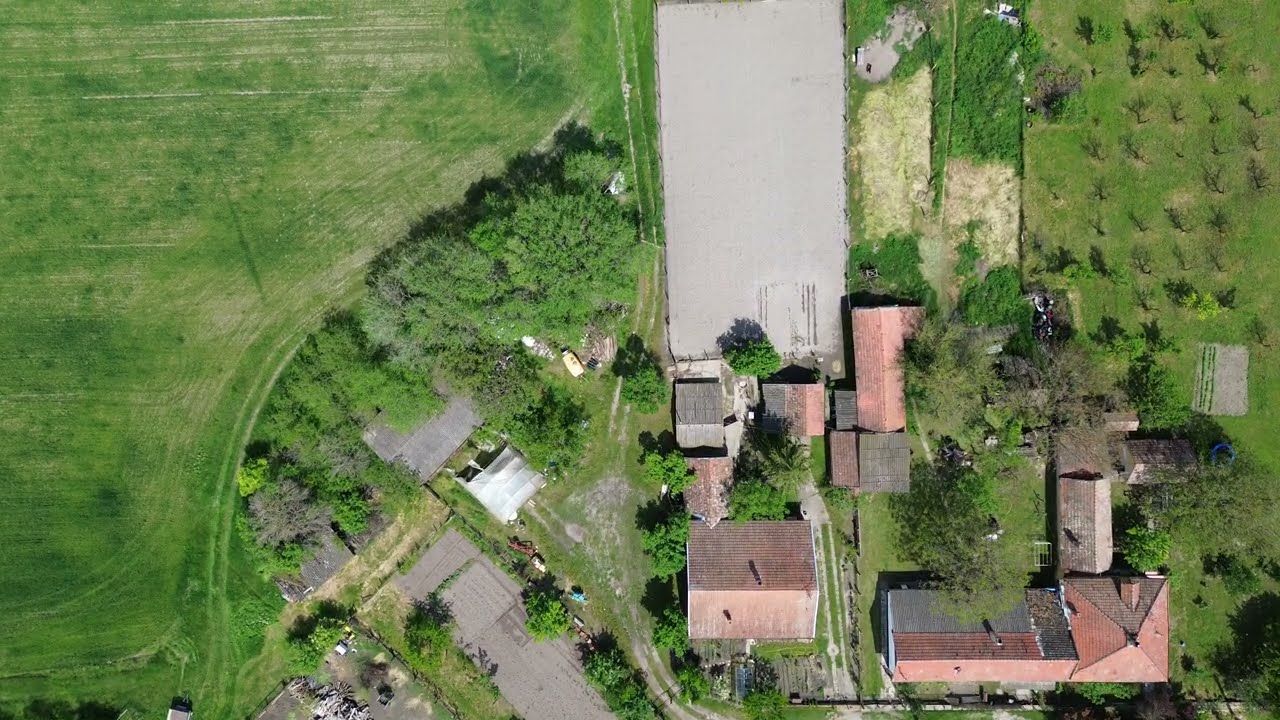An aerial photograph captures a vivid scene of rural acreage dominated by bright green farmland. The landscape, viewed from directly overhead, primarily showcases expanses of grass and various trees. On the left side, there are mature deciduous trees, while the upper right corner features a grid-like pattern of smaller, leafless trees, possibly an orchard. Scattered throughout the greenery are several buildings with distinctive reddish-brown and gray roofs, some with triangular steeple tops, others more rectangular in shape. 

Prominently, a large silver-gray rectangle is visible, which might be a significant structure or a parking area. Surrounding this central area are smaller parking lots, some vehicles, and possibly farm equipment. The central part of the photograph includes fenced enclosures, perhaps containing barns or animal housing, with the fencing suggesting an area intended for exercising animals like horses. 

Clumps of trees appear in the lower left, while fields of grass, with visible tractor-induced streaks, stretch across the upper left. Additional notable features include stone slabs resembling wide driveways and scattered piles that could be supplies or refuse. The right side is marked by more spaced-out trees, reinforcing the orchard appearance, along with the occasional sighting of farm vehicles and a giant woodpile. This intricate and detailed depiction of a rural setting effectively combines varying elements of nature and human habitation.